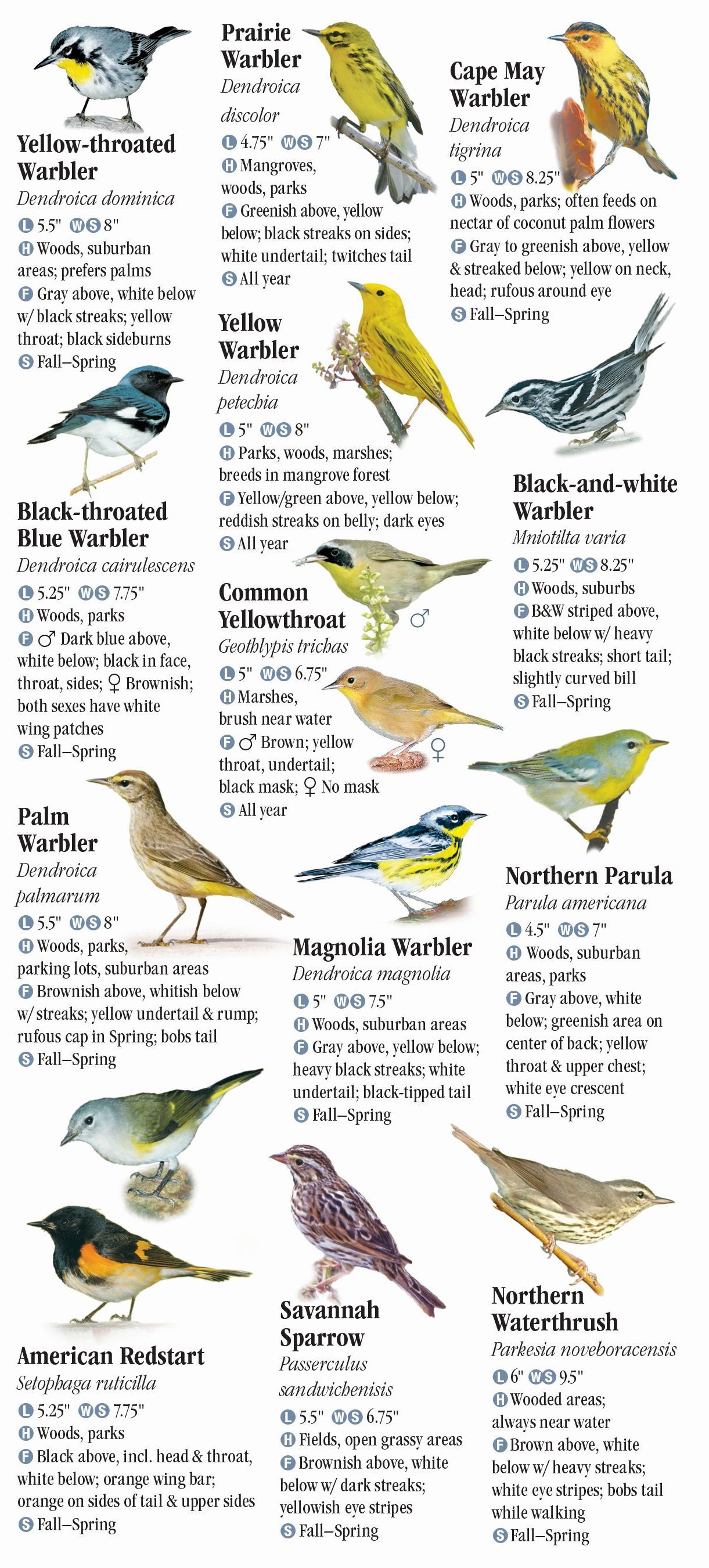The image is a detailed page from an ornithology guide, featuring realistic color illustrations of approximately 15 different songbirds on a white background. Each bird is accompanied by its name in bold lettering, followed by a lighter font blurb providing key information such as size, habitat, and seasonal sighting details. The birds are arranged in three columns. The first column features a Yellow-throated Warbler, Black-throated Blue Warbler, Palm Warbler, and American Redstart. The second column includes a Prairie Warbler, Yellow Warbler, Common Yellowthroat (both male and female), Magnolia Warbler, and Savannah Sparrow. The third column displays a Cape May Warbler, Black-and-white Warbler, Northern Parula Warbler, and Northern Waterthrush. The array of birds includes species with striking blue, yellow, orange, green, and brown plumage, emphasizing warblers and a few other types like the Northern Waterthrush. The guide is reminiscent of an Audubon field guide, providing enthusiasts with a comprehensive identification and information resource.